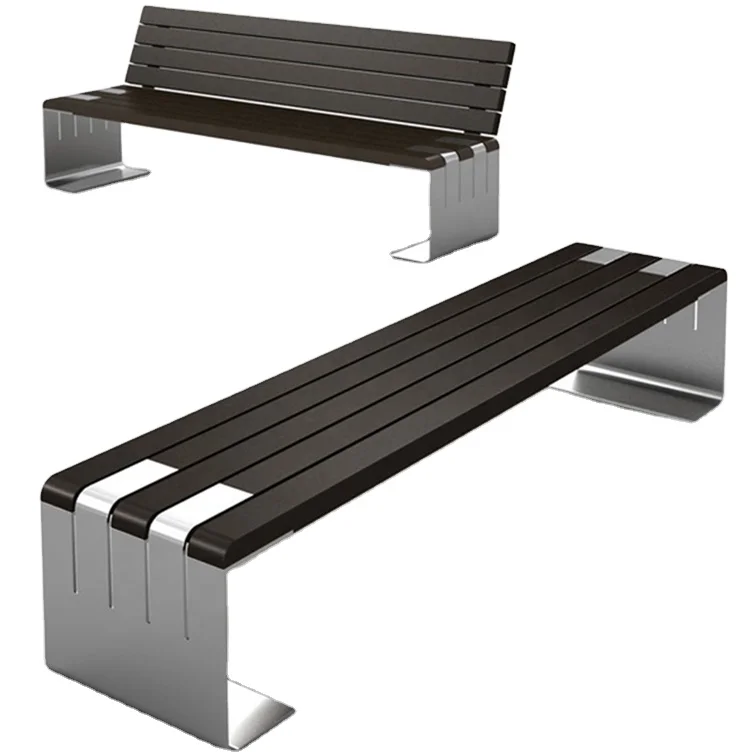This product photograph showcases a pair of robust, industrial-style benches designed for outdoor use, such as at bus stops or parks. Both benches feature a sleek, modern aesthetic with a slightly futuristic touch. The bench positioned on the upper left has a distinctive black slat appearance, resembling wood but actually crafted from durable black metal. It is supported by wide, silver legs made from chrome or brushed stainless steel, which run the length of the bench and curve underneath to provide stability. This bench offers both a seat and a backrest, each composed of five dark brown or black slatted panels.

The bench located on the lower right matches the first in design but lacks a backrest, presenting a more streamlined profile. It features the same sturdy silver legs extending to the ground. The background is white or transparent, emphasizing the benches' modern, minimalist design. Although striking in appearance, with their metallic sheen and sleek lines, these benches prioritize durability over comfort, presenting a practical seating solution for public spaces.